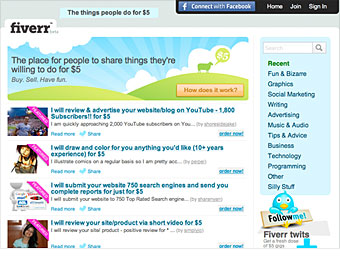Here is a detailed, cleaned-up descriptive caption for the image:

---

This image is a small screenshot depicting an early iteration of the Fiverr website, characterized by a dated design. Along the top section of the website, the header features a light gray background with a light blue chat bubble containing black text that reads, "The things people do for $5." To the top right, there's a menu on a dark background offering options such as "Connect to Facebook," represented by a rectangular button, followed by "Home," "Join," and "Sign In" in white letters.

Below this header, and to the left, is the Fiverr logo presented in black serif letters that pop up like a tab. Beneath the logo, there is an image with the text, "The place for people to share things they're willing to do for $5," along with the phrases "Buy, Sell, Have Fun." This text is enclosed within an illustrated picture featuring two green hills, one of which has a green silhouette of a sheep with a chat bubble saying "$5." In the background, illustrated clouds and sun rays add to the whimsical design. At the bottom right of this image, the text reads, "How does it work?"

On the right side, a sidebar presents four rows of articles. Each row includes a thumbnail image with a purple ribbon at the top right corner, followed by a title, subheading text, and various links. The first thumbnail appears to be an image of a man against a blue sky or stadium, with the accompanying title reading, "I will review and advertise your website blog on YouTube. 1,800 subscribers for $5." The second row features a thumbnail that looks like a picture of a woman and includes the title, "I will draw and color for you anything you like, 10+ years experience for $5." Two more rows follow in the same format.

Beneath these rows, a side menu with a white background features a blue rectangular section at the top, containing a search bar labeled "Recent." Categories such as "Fun and Bizarre," "Graphics," "Social Marketing," "Writing," "Advertising," "Music and Audio" are listed below. At the very bottom, in the bottom right corner, there is an old Twitter graphic that reads "Follow me," picturing a digital blue bird embracing a sign that says "Fiverr Twits."

---